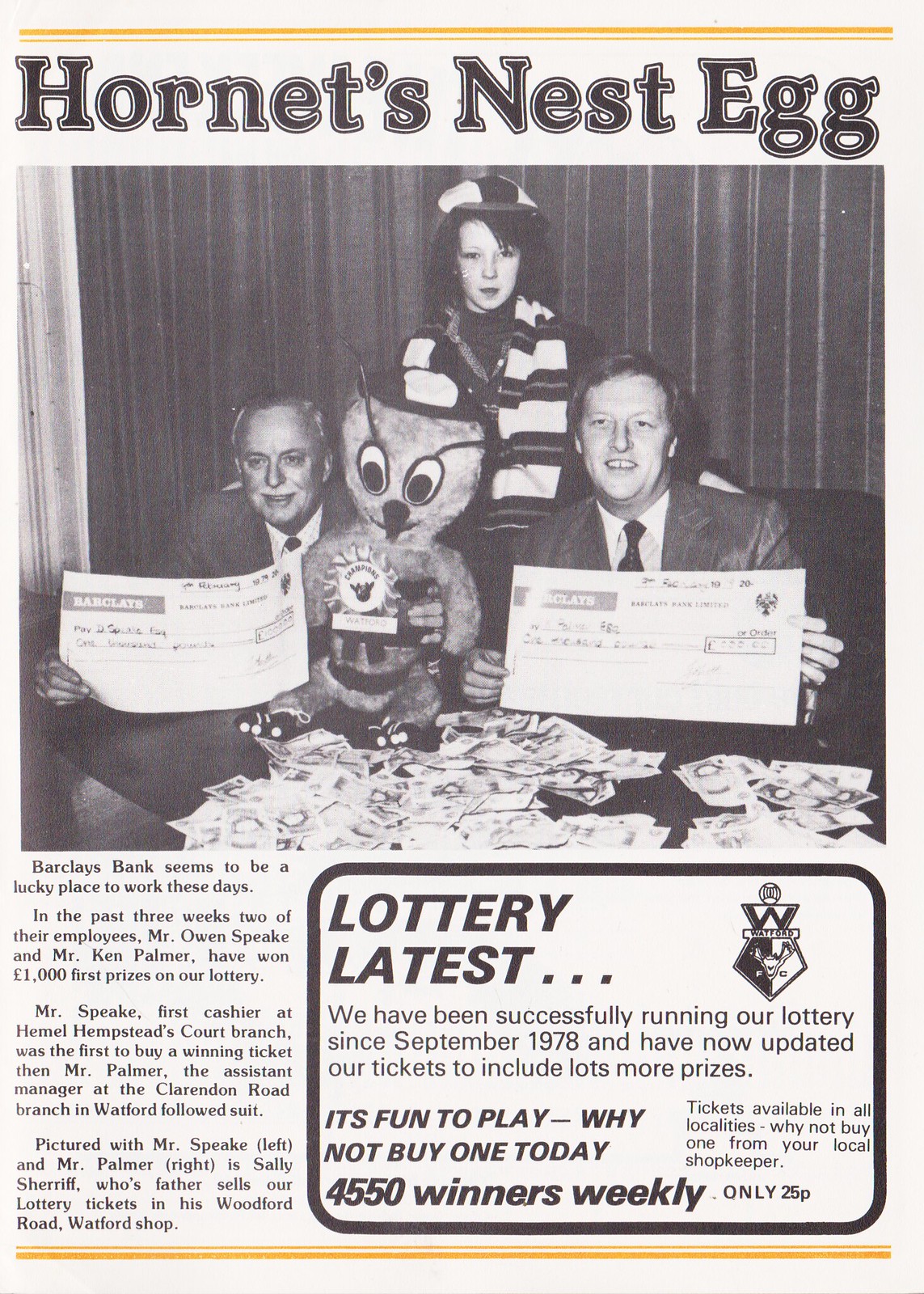This vertically oriented newspaper clipping features a prominent title at the top, "Hornet's Nest Egg," flanked by two horizontal yellow lines—the top line being notably thicker. Below the title, the main body of the clipping showcases a large black-and-white photograph depicting two older men seated at a table, each holding oversized paper checks, and a young woman standing behind them. The woman, who has long hair and is wearing a striped scarf with a matching hat, appears stoic while the men are smiling. Nestled between the men is a plush toy, resembling a hornet or mascot, holding a trophy. Spread across the table in front of them is a scattering of cash. 

The text below the image provides context: "Barclays Bank seems to be a lucky place to work these days. In the past three weeks, two of their employees, Mr. Owen Speak and Mr. Ken Palmer, have won 1,000 pounds, first prize in our lottery. Mr. Speak, first cashier at Hemel Hempstead's Court Branch, was the first to buy a winning ticket, followed by Mr. Palmer, the assistant manager at the Clarendon Road branch in Watford. Pictured with Mr. Speak (left) and Mr. Palmer (right) is Sally Sheriff, whose father sells our lottery tickets in his Woodford Road, Watford shop."

The clipping concludes with a section labeled "Lottery Latest" in bold text, encased in a border. It reads, "We have been successfully running our lottery since September 1978 and have now updated our tickets to include lots more prizes. It's fun to play—why not buy one today? 4,550 winners weekly. Tickets available in all localities. Why not buy one from your local shopkeeper? Only 25p."